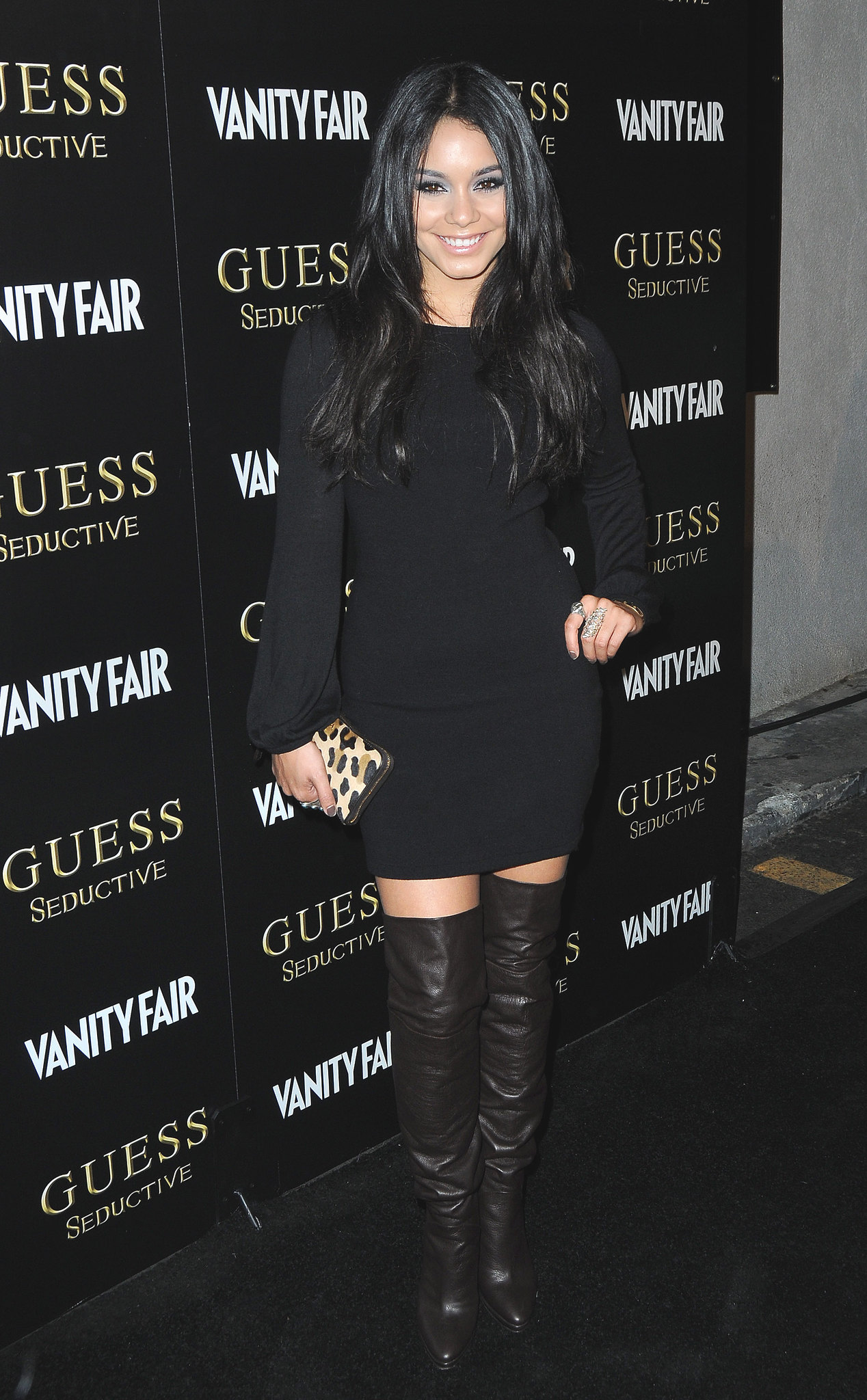The photograph features an attractive young woman, presumably a model or celebrity, posing at a fashion event or lounge indoors. She is standing in front of a backdrop repetitively printed with "Vanity Fair" and "Guess Seductive," likely indicating the event's sponsors. The woman gazes directly into the camera with a smile. She has long, dark hair cascading over her shoulder and is dressed in a form-fitting black dress that reaches mid-thigh. Complementing her outfit, she wears thigh-length leather boots. She accessorizes her ensemble with a tiny leopard print purse, adding a touch of flair to her sophisticated look.